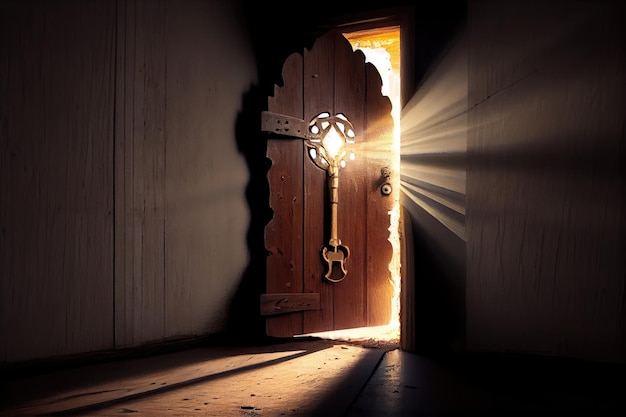The image depicts the interior view of a medieval-style room, focusing on a wooden front door made of dark brown panels. The room is enveloped in darkness, enhancing the contrast with the bright, golden-yellow light streaming in through both the small window in the door and the narrow opening as the door slightly ajar. This light creates a glowing effect that highlights intricate wood engravings around the window, featuring vine and diamond patterns. The door's centerpiece resembles a keyhole shape, adding to the rustic charm, and a gold door knocker hangs prominently. The scallop-shaped, rich dark brown walls and dark wooden floors contribute to the overall medieval, almost 'hobbit-like' atmosphere, reminiscent of an environment from Lord of the Rings. The vibrant rays illuminate the room’s timeless wooden aesthetic, creating a captivating interplay of light and shadow.